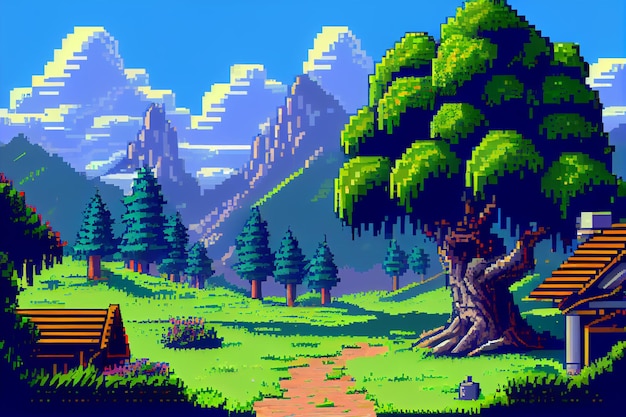The image, reminiscent of 1990s pixel art style, portrays a pixelated outdoor environment with a serene landscape that feels like it belongs in an 8-bit computer game. Dominated by tiny squares forming intricate details, the scene is set under a clear blue sky with sporadic white clouds and sunlight shining on the surroundings. The background showcases a tall, rocky mountain range with hues of green and purple, topped prominently by pine trees. Towards the middle-bottom of the image, a small, dark path winds its way through a vast green field dotted with various conical-shaped trees and foliage. 

On the right-hand side, there's a massive, ancient oak tree, its thick trunk supporting a lush canopy of green leaves, emphasizing its age and grandeur. Nearby, partially cropped, is a house with a triangular roof, brown in pattern, standing out with visible pillars and an entrance leading to a green lawn below. To the left, partially hidden by foliage, another triangular-roofed structure, resembling a small shed, peeks into view. This captivating pixel art landscape, devoid of any textual elements, invites viewers into its tranquil, digital world.